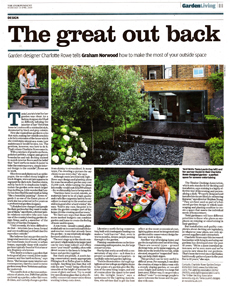The newspaper article titled "The Great Outback" features bold headings, with "Garden Living" prominently displayed, the word "Garden" in a bolder font compared to "Living." The article appears on page 11. It discusses garden design, mentioning designers Charlotte Rome and possibly another designer named Belk. Boldly highlighted is Graham Norwood's section, "How to Make the Most of Your Outside Space." Accompanying the text are several images: a picture of a woman and a man at a picnic table, a photograph of a house, and a family eating together at a bench.